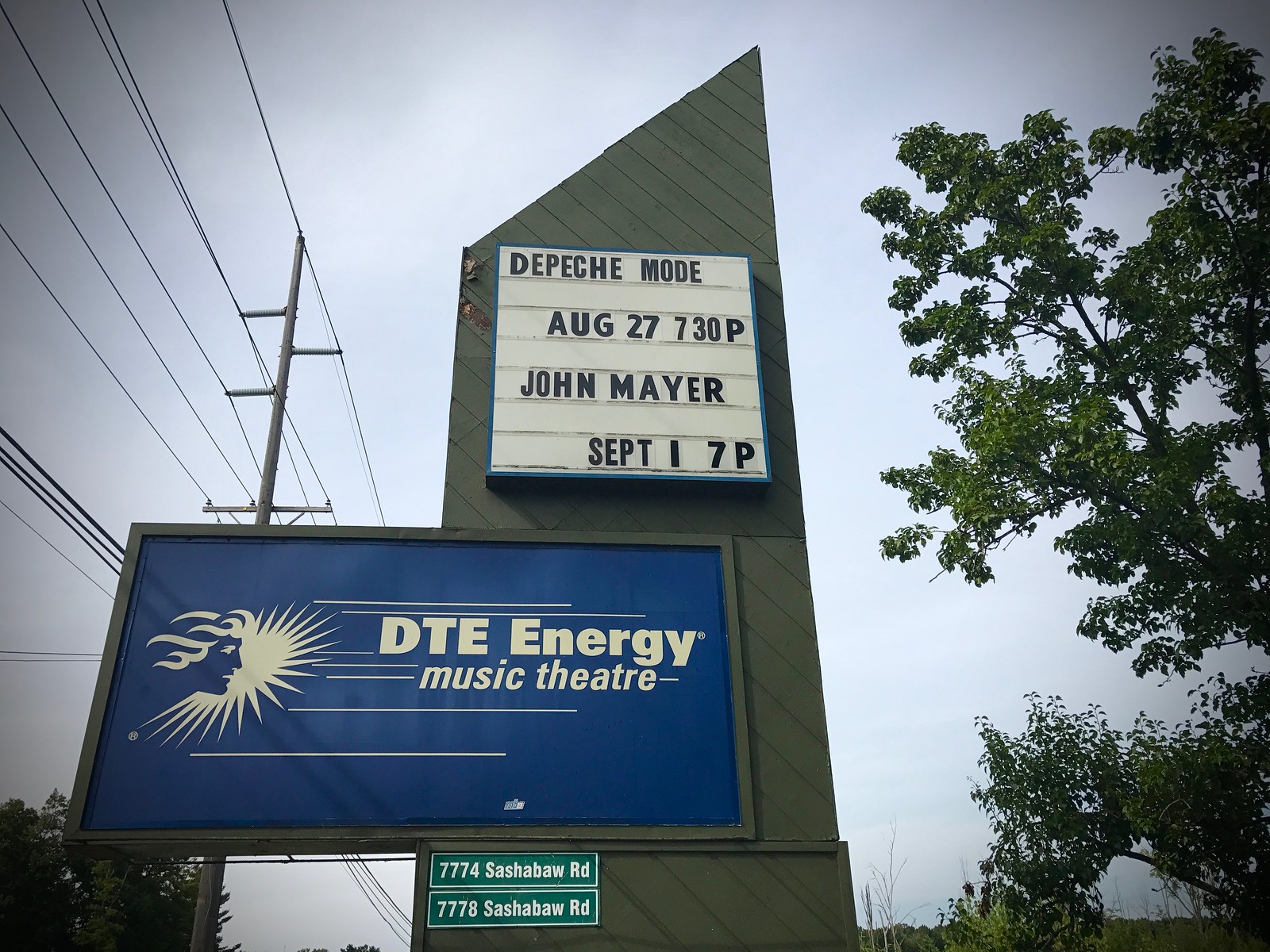In the center of the image, there is a tall, monolithic wooden structure with a pointed top, prominently featuring customizable, slatted white signage. This venue advertisement lists upcoming musical acts, with black text reading "Depeche Mode, August 27th, 7:30 p.m." and "John Mayer, September 1st, 7 p.m." Below this, a bold blue billboard displays "DTE Energy Music Theater," indicating the venue's name. Also detailed on the structure are two street addresses: 7774 Sashaba Road and 7778 Sashaba Road. The setting appears to be outdoors during the day, with visible power lines in the top left, a backdrop of green trees to the right, and a sky featuring hues of gray, blue, white, and touches of brown.